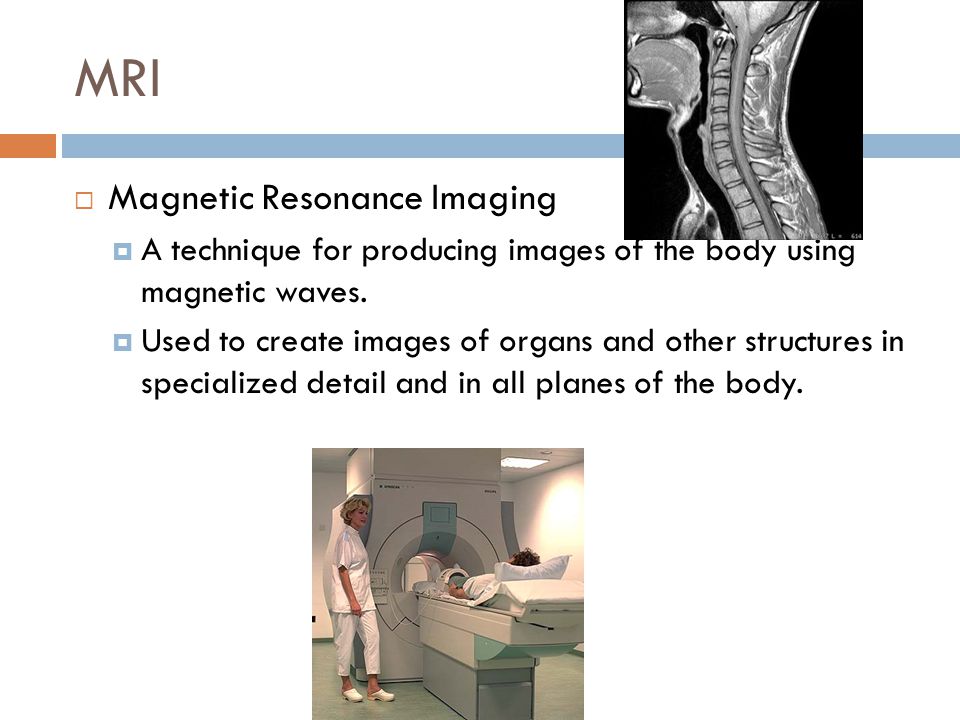The image is a detailed infographic with a white background, prominently featuring information and visuals related to MRI (Magnetic Resonance Imaging). The top part of the infographic is anchored by the title "MRI" in bold text to the left, atop an orange rectangular section and a blue horizontal line. Below the title, there's an explanatory text in bullet points that reads: "Magnetic Resonance Imaging, a technique for producing images of the body using magnetic waves. Used to create images of organs and other structures in specialized detail and in all planes of the body."

On the right-hand side, overlaying the blue line, there is a cross-sectional graphic resembling an X-ray or MRI scan, depicting the neck and head including the vertebrae, esophagus, and spinal cord, which appears to be a detailed cadaver cross-section.

Below this section, there's a photograph featuring a woman dressed in white, standing beside a large MRI machine within a medical or healthcare setting. A patient is lying on the MRI table with their head on a pillow, positioned to enter the machine for imaging. The overall color scheme includes brown, orange, blue, black, gray, and yellow, contributing to a visually informative presentation that emphasizes the medical and educational context of MRI technology.